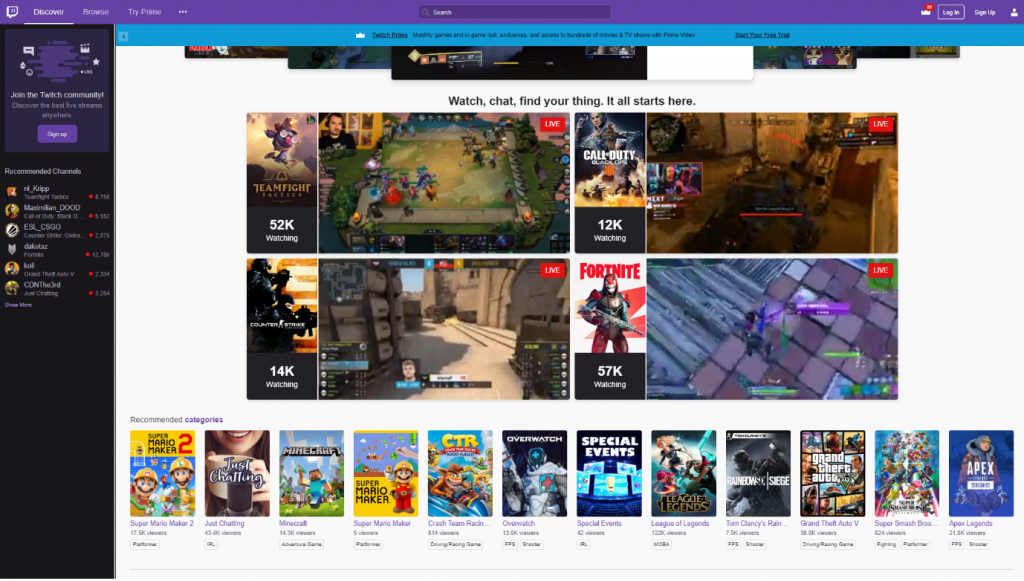A vibrant preview screen for an online video game platform is displayed. At the bottom, a row of video game cover images allows users to select different titles, akin to a menu of DVDs. Four popular games are highlighted: Team Fight, Call of Duty, Fortnite, and one other title, whose name is unclear due to the small and blurry font. 

In the center are four interactive squares, each presenting a snippet of gameplay. A small preview in the corner of each square shows a live player in action, while the main view provides a detailed screenshot of the game. Accompanying each screenshot is the number of current viewers: 52K, 12K, 14K, and 57K respectively, indicating the popularity of each game. 

Above these previews, a banner reads: "Watch, Chat, and Find Your Thing. It All Starts Here," suggesting users can engage with the platform by observing gameplay, participating in chats, and possibly even joining the games themselves. The overall interface hints at a dynamic, community-driven gaming environment where users can immerse themselves in both playing and viewing experiences.